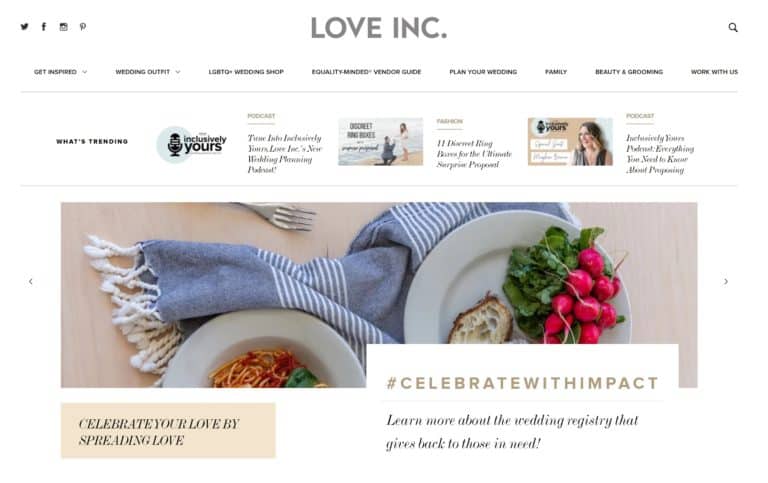The image portrays a webpage from the website "Love Incorporated" (spelled in all capital letters: L-O-V-E I-N-C), with the name displayed in grey text at the center top of the image. To the far left of the "Love Inc" logo, there are social media icons for Twitter, Facebook, and another unidentified platform. Adjacent to the logo on the right side is a magnifying glass icon, symbolizing a search function.

Beneath the logo, a navigation bar lists several categories. Visible are "Get Approved Wedding Outfit" and an incomplete category name mentioning "Wedding Shop." There are five additional categories, but the text is too small to be legible.

Directly below the category bar is a rectangular section labeled "What's Trending Exclusively Yours," followed by brief, unclear text and an image for another category.

Further down, the section titled "Celebrate with Impact" showcases a photograph featuring a table set with two plated entrees: one of spaghetti and the other consisting of bread and radishes. The caption "Celebrate with Impact" (formatted as a hashtag: #CelebrateWithImpact) follows, along with a call-to-action: "Learn more about the wedding industry that gives back to those in need!"